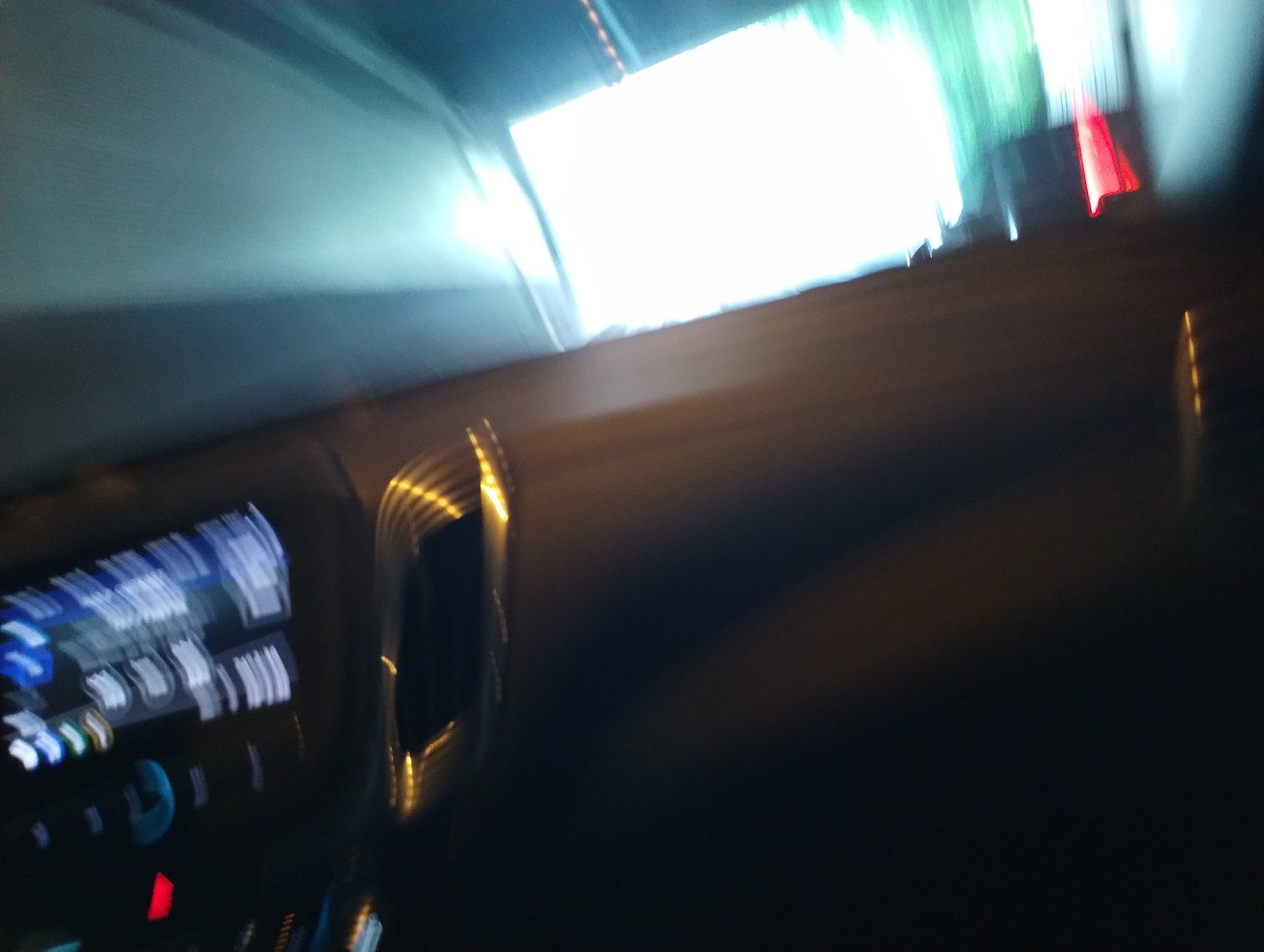This extremely blurry photograph captures the interior of a car from the perspective of the passenger seat. Central to the image is the dashboard featuring various illuminated lights, possibly from the GPS or radio system. These lights display numbers but are indiscernible due to the blurriness. The dashboard, colored in dark gray, is highlighted by textured, silver-tinged vents, an effect likely intensified by the camera's motion. In the lower right corner of the image, the car's interior fades into darkness and blur. Through the windshield, a reflection of a red triangle appears in the right corner, suggesting possible dashboard indicators or external lighting. The car seems to be parked inside a dimly lit garage, with faint outlines of dark concrete walls and ceiling visible amidst the blur. A large, square-shaped light source is positioned almost centrally, adding to the hazy ambiance of this motion-captured scene.